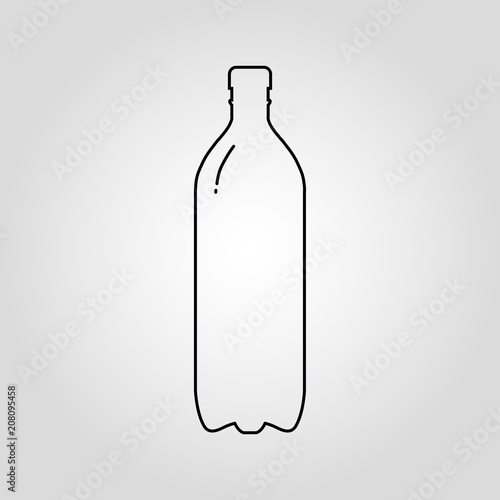The image depicts a simplified, computer-generated drawing of a tall plastic bottle. Rendered with black lines, the bottle features an elongated body and a narrow cap, with an additional curved line on the upper left side adding a slight 3D effect. At the base, the bottle rests on three points. The background is a muted grayish-white or cream color. There are multiple Adobe Stock watermarks embedded in the background. Notably, in the bottom left corner, there is black text rotated 90 degrees counterclockwise that reads "Adobe Stock" and "number 208095458."